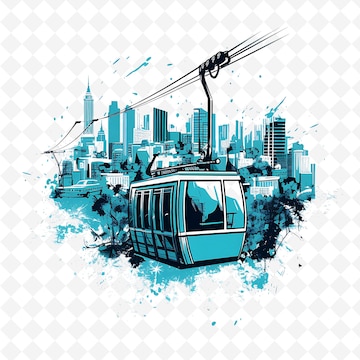The image is a cartoon drawing dominated by shades of black, blue, white, and aqua. Central to the illustration is a blue aerial cable car with large windows and side doors, connected to black wires and a metal pole. The foreground highlights the cable car, which appears much larger, suggesting it is moving across the scene. In the distance, a city skyline—likely New York City due to the presence of a building resembling the Empire State Building—can be faintly seen, along with other skyscrapers and a few trees scattered throughout. The background and edges of the image feature a checkerboard pattern of white and dark squares, adding an artistic and unique frame to the drawing. The overall composition merges linear architectural elements with fluid, paint-splashed borders, emphasizing the contrast between the structured cityscape and the more abstract edge detailing.